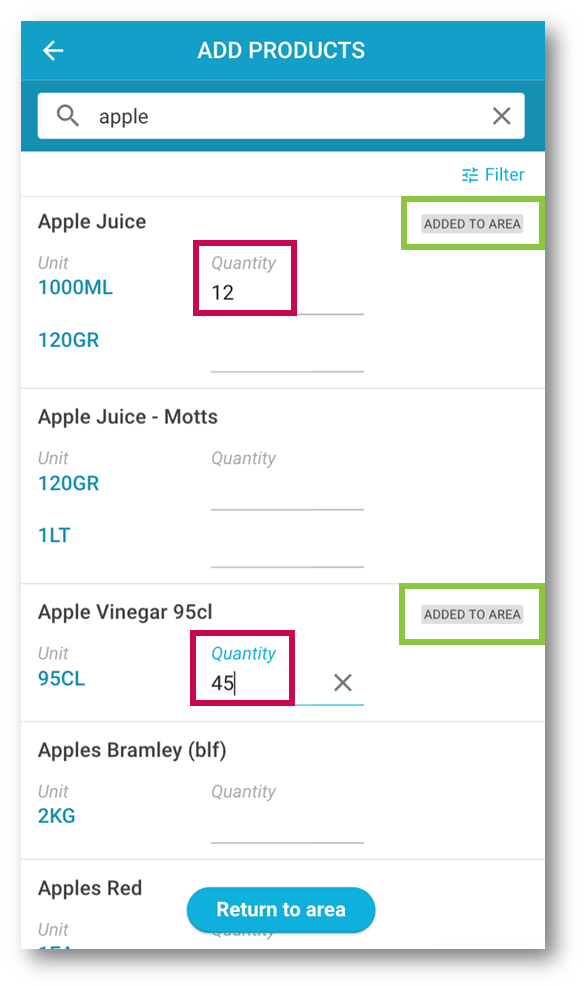The screenshot from a cell phone displays a user interface for adding products. The interface is predominantly organized into a structured list with several sections and features:

At the top of the screen, a blue bar spans the width of the interface. Positioned on the left side of the blue bar is a white left-facing arrow. Centrally located within the blue bar, white text reads "Add Products." Directly below the blue bar, there is a search bar. The placeholder text within the search bar says "Apple." On the right side of the search bar, there is an 'X' icon. Adjacent to the right end of the search bar, a blue button labeled "Filter" is visible.

Moving down, the first product listed is "Apple Juice," written in bold black letters on the left. Below this, "Unit 1000 ML" is displayed in blue text. To the right of these details, there is a red box containing the word "Quantity" in gray, accompanied by the number "12" in black. Further below "Apple Juice" on the left, "120GR" is marked in blue, with an empty area to its right.

The next listing shows "Apple Juice/Motts" in bold black letters. Below it, the word "Unit" appears in gray, followed by "120GR" in blue. To the right of this, a header labeled "Quantity" is seen with a blank space below it. Further, beneath this section on the left, "1LT" is indicated in blue, with an adjacent empty space to the right.

Continuing down, "Apple Vinegar 95CL" is written in bold black letters, with a green box to its right containing "Added to Area" in gray. On the left, "Unit" is presented in gray, with "95CL" in blue text next to it. To the right, "Quantity" is displayed in blue, alongside "45" in black, encased in a red box. To the right of this quantity box, a gray 'X' is visible.

Below this, "Apple's Bramley BLF" is displayed in bold black letters. Underneath, "Unit" appears in gray, with "2KG" right below in blue. To the right, the word "Quantity" is in gray, followed by a blank space beneath it.

At the bottom, the listing titled "Apple's Red" is in bold black letters. Underneath, "Unit" is noted in gray text, but the remainder is cut off in the screenshot. To the right, there is a blue button labeled "Return to Area" with white text inside it.